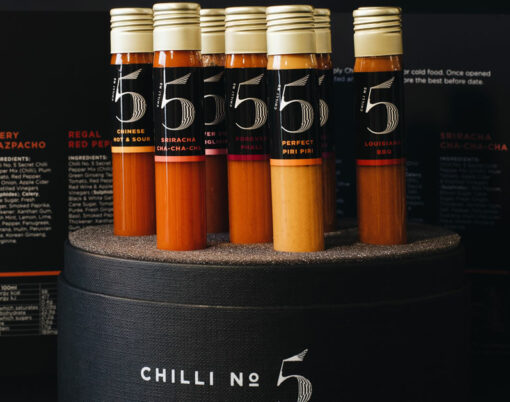The image showcases a professionally taken photograph intended for the brand "Chili No. 5." Set against a predominantly dark background with white and red text, the focal point is a black cylindrical container with a gray top surface, prominently labeled "Chili No. 5" in white lettering along its base. Inside the container are seven vials standing upright, each with a gold screw cap and a black label featuring a large number '5'. The vials contain various chili sauces, ranging in color from tan to deep red. Each vial is meticulously labeled, detailing the type of sauce such as "Sriracha, Cha-Cha-Cha," "Chinese, Hot and Sour," and "Perfect, Piri-Piri," among others. The background includes additional, yet unclear, text and serves to highlight the sophisticated aesthetic of the brand.